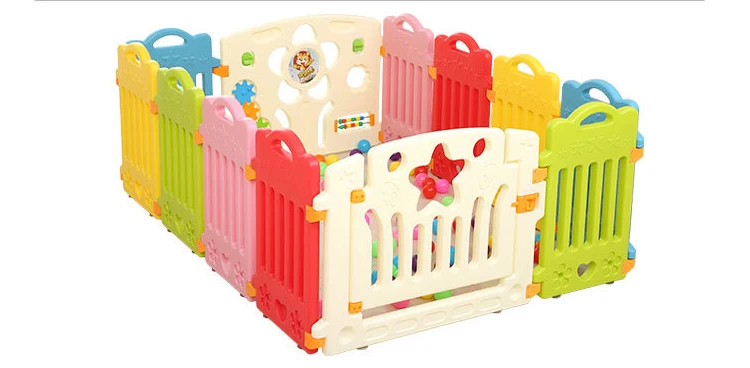The image depicts a colorful rectangular playpen designed for a small child or toddler. The playpen is enclosed by interconnected plastic panels of various colors, including red, pink, green, yellow, and blue. The front features a white gate with a star-shaped cutout, flanked by a green panel to the left and a red panel to the right, followed by pink, green, and yellow panels. Inside the pen, there's a vibrant array of rainbow-colored balls and various toys, including turning gears and flipping knobs on the back panels. Additionally, the back features another large, white panel adorned with a cartoon cat inside a flower, providing more playful interaction points. The setup is characterized by its colorful, engaging design, aimed at keeping a child entertained within a safely enclosed area.